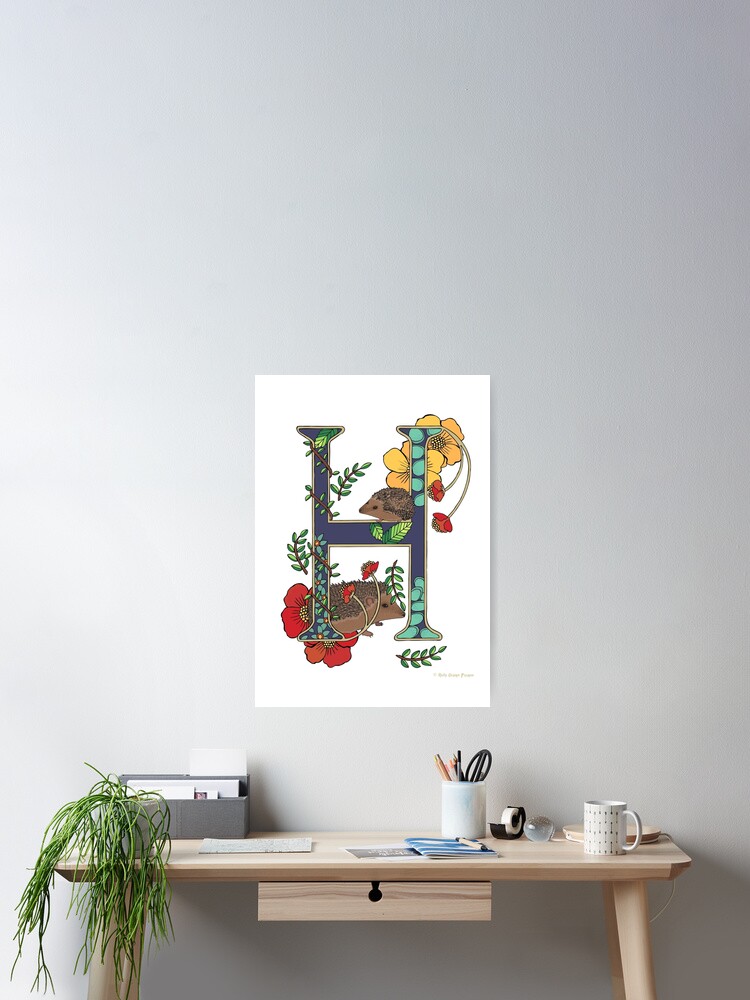The photograph features a small, light wood desk set against a gray background wall that prominently displays a white poster adorned with a large, multicolored letter "H." The "H" is decorated with vibrant purple and blue shades, surrounded by red and yellow flowers and green vines. The minimalist wooden desk, supported by four legs, has a central drawer for storage. On the desktop's left side sits a potted fern draping over the edge, with a gray box behind it containing visible papers. A Pixar-style adjustable lamp with a white container at the top is positioned on the desk's right side. Nearby, a white mug holds scissors, pens, and pencils, while a roll of tape and some scattered papers add to the workspace's functionality. A brown tray and a white coffee cup complete the organized yet busy scene.